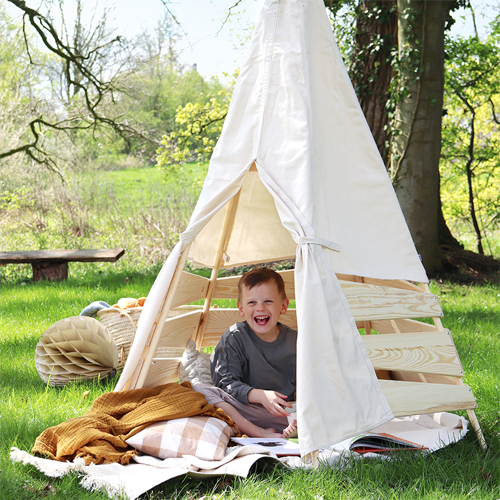In a serene, grassy yard, a young boy with dark hair and a gray long-sleeve shirt beams with laughter while sitting inside a charming teepee. The teepee, resembling a cone-shaped structure, is crafted from wooden poles draped with an off-white cloth, offering an inviting and cozy retreat. Surrounding the boy are various comforts: a red and white striped pillow, a tan blanket, and a book, all arranged neatly inside the teepee. To the left of this delightful scene is a handmade wooden bench fashioned from a couple of round, unsplit logs topped with a rectangular wooden plank, adding to the rustic atmosphere. Behind the boy, the backdrop features a lush lawn adorned with trees, some bearing blossoms and some with bare branches, enhancing the natural setting. It's a sunny day, and the boy’s radiant smile captures the pure joy of this tranquil outdoor moment.